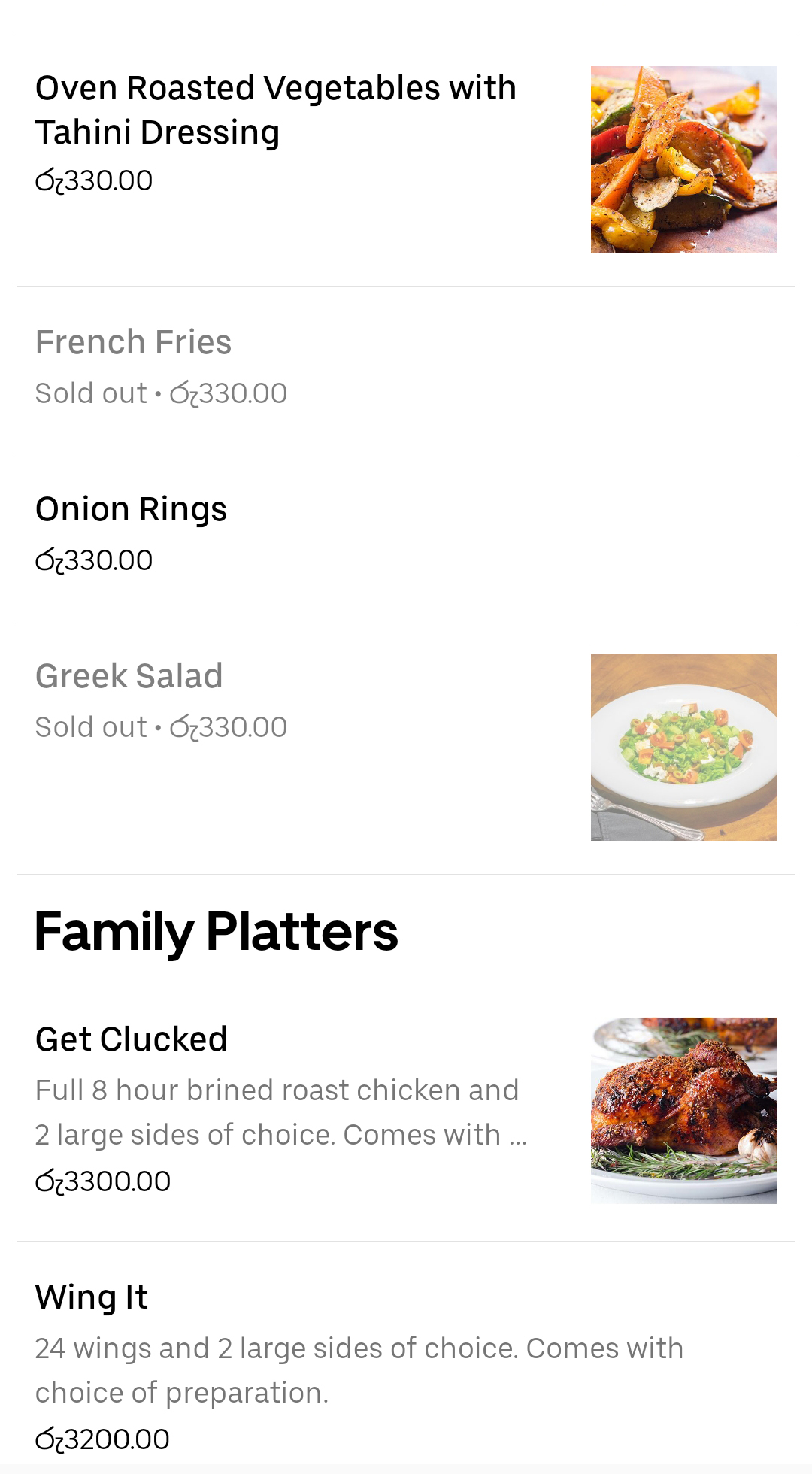Here's a cleaned-up and detailed descriptive caption for the described image:

"A screenshot taken from a restaurant's online menu displaying food items priced in an unfamiliar currency. At the top of the menu is 'Oven Roasted Vegetables with Tahini Dressing,' listed at 330 (currency symbol unclear). A corresponding image shows a colorful assortment of seasoned, grilled vegetables. Following that are 'French Fries' and 'Onion Rings,' both without accompanying photos. 'Greek Salad' is pictured but marked as 'Sold Out.' 

A separate section titled 'Family Platters' includes 'Get Clucked,' featuring a fully roasted chicken brined for eight hours, plus two large sides. The description is partially cut off, but a prominent image of the juicy roasted chicken is displayed. The final item listed is 'Wing It,' which offers 24 wings and two large sides but lacks an image. Items in this section are notably more expensive, roughly ten times the cost of individual dishes. The menu has a clean design with a white background and black text, giving it a sophisticated yet pricey appearance."